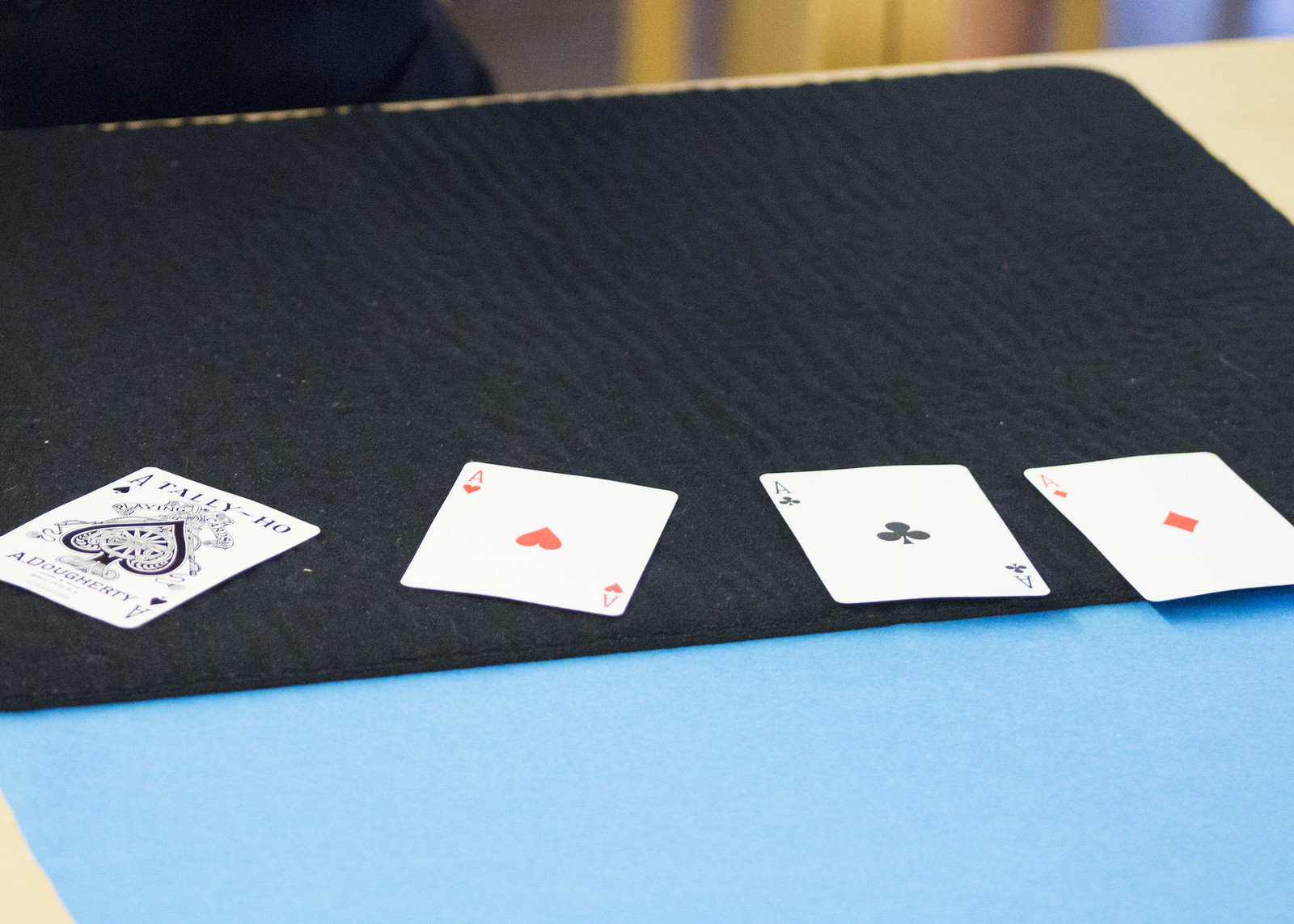In this horizontally oriented photograph, a tranquil and organized gaming scene is depicted. The focal point is a table with a smooth, baby blue surface, devoid of any texture. Dominating the center of this table is a fluffy, black rectangular mat with elegantly rounded edges, providing a contrasting backdrop to the cards placed upon it.

Positioned on the mat, impeccably aligned in a row from left to right, are four playing cards, all face up and each one an ace. The sequence begins with the Ace of Spades, featuring a white background and bold black spade symbol. Next in line is the Ace of Hearts, immediately noticeable with its striking red heart on a white background. Following this is the Ace of Clubs, characterized by the classic black club symbol against the white backdrop. Concluding the sequence is the Ace of Diamonds, displaying its vibrant red diamond shape on a white background.

This meticulously arranged setting, highlighted by the smooth blue table and the cushioned black mat, emphasizes the prominence and uniformity of the aces, creating a visually appealing and detailed composition.